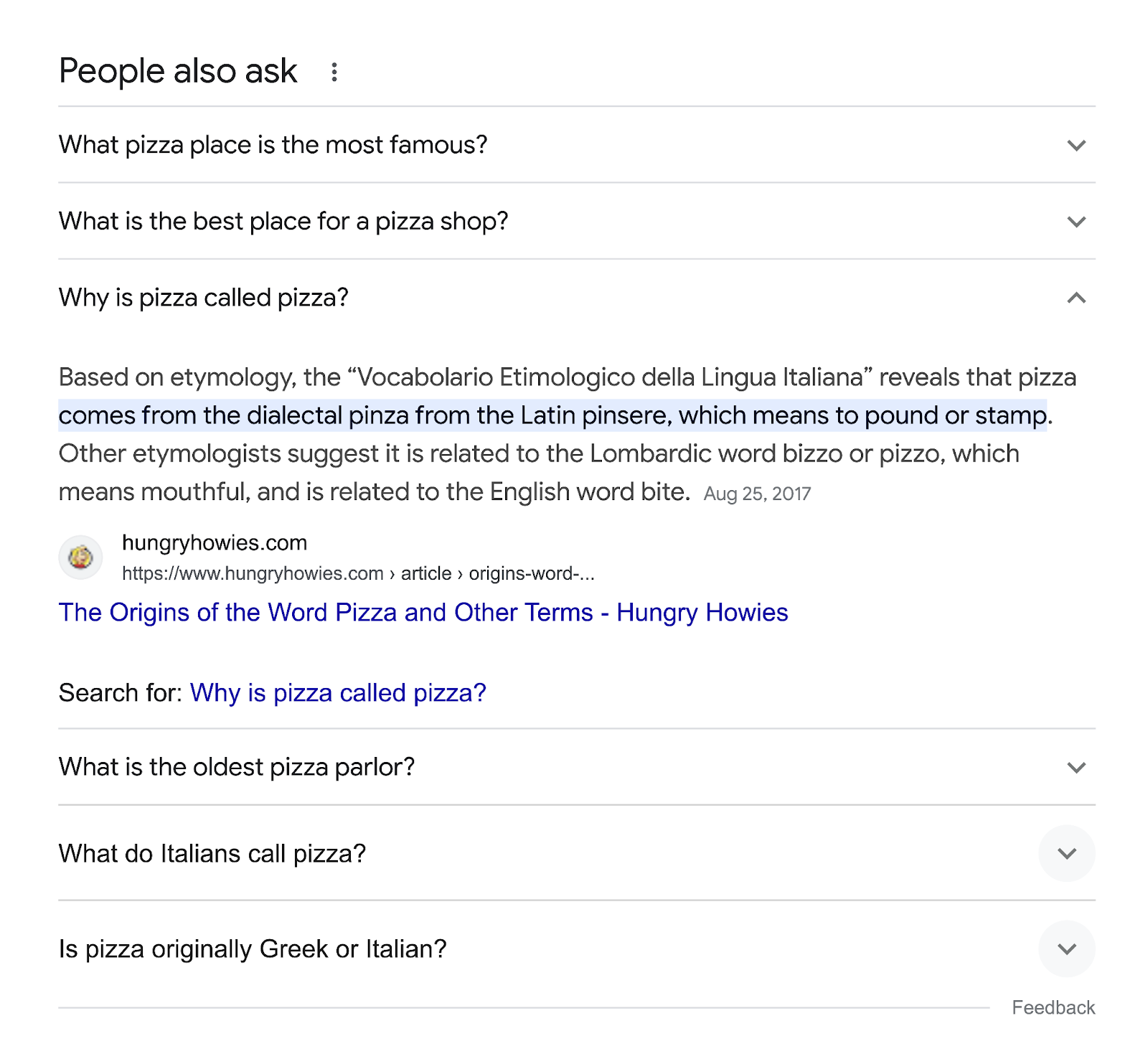In the image, the top part displays a Google search bar with the query "people who ask." Below it, three questions are listed: 
1. "What pizza place is the most famous?"
2. "What is the best place for a pizza shop?"
3. "Why is pizza called pizza?"

Following these questions, there is a detailed explanation about the etymology of the word "pizza." The text, enclosed in quotation marks, reads: "Based on Etymology, the 'Vocabulario Etymologico della lingua italiana' reveals that 'pizza' comes from the dialectal 'Pinsa' from the Latin 'pincere,' which means to pound or stamp. Other etymologists suggest it is related to the Lombardic word 'beasel' or 'beisel,' which means mouthful and is related to the English word 'bite.'"

Beneath this explanation, a website link to "hungryhowies.com" is shown. The URL is followed by the title in blue: "The origins of the word pizza and other terms - Hungry Howie's." 

Below this title, there is a prompt suggesting a follow-up search: "Search for why is pizza called pizza?"